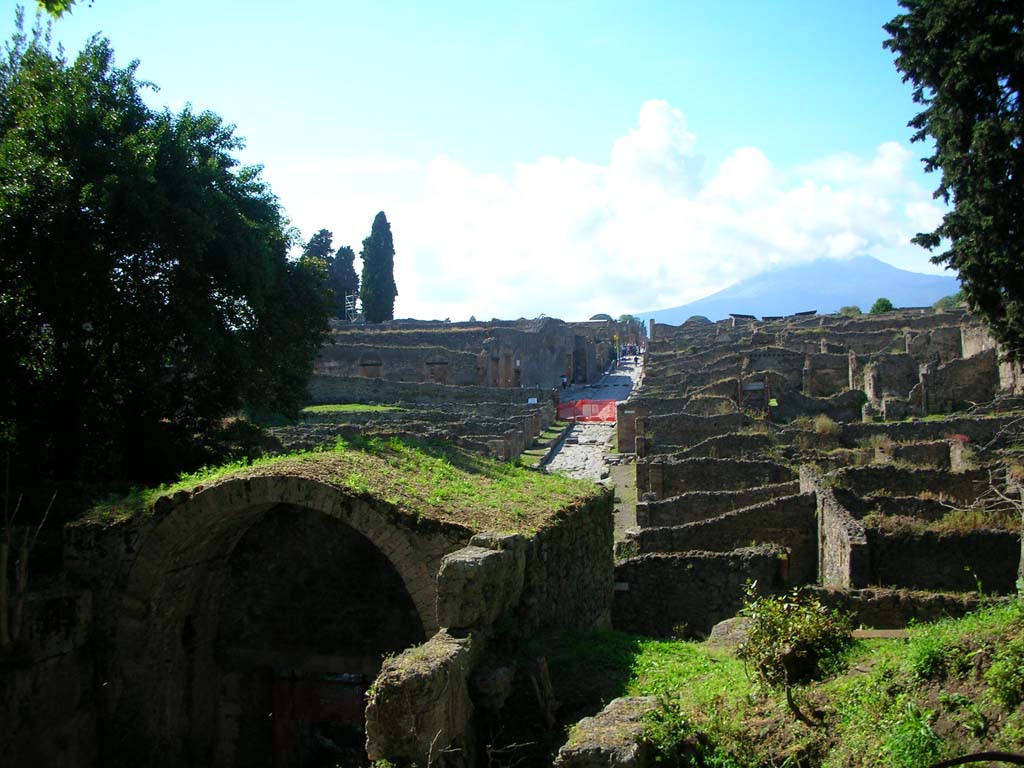The photograph, taken outdoors during the daytime, captures an expansive scene of ancient ruins nestled on a hillside beneath a light blue sky dotted with clouds. The ruins, constructed from light gray stone, are interspersed with moss and small plants. At the forefront stands a moss-covered archway leading through a tunnel-like opening, flanked by trees. Beyond this arch, the remaining low stone walls and half-destroyed structures stretch across the landscape, forming a complex of what were once houses or communal buildings. A broad pathway, possibly an original cobblestone road, runs prominently through the middle of the site. In the background, framed by greenery and trees, a distant volcanic peak rises, partially shrouded in clouds, adding a dramatic touch to the historical ambiance. Tourists can be seen exploring the site, walking along the main pathway, while colorful signs and banners punctuate the scene, hinting at modern efforts to guide and inform visitors about this ancient town.